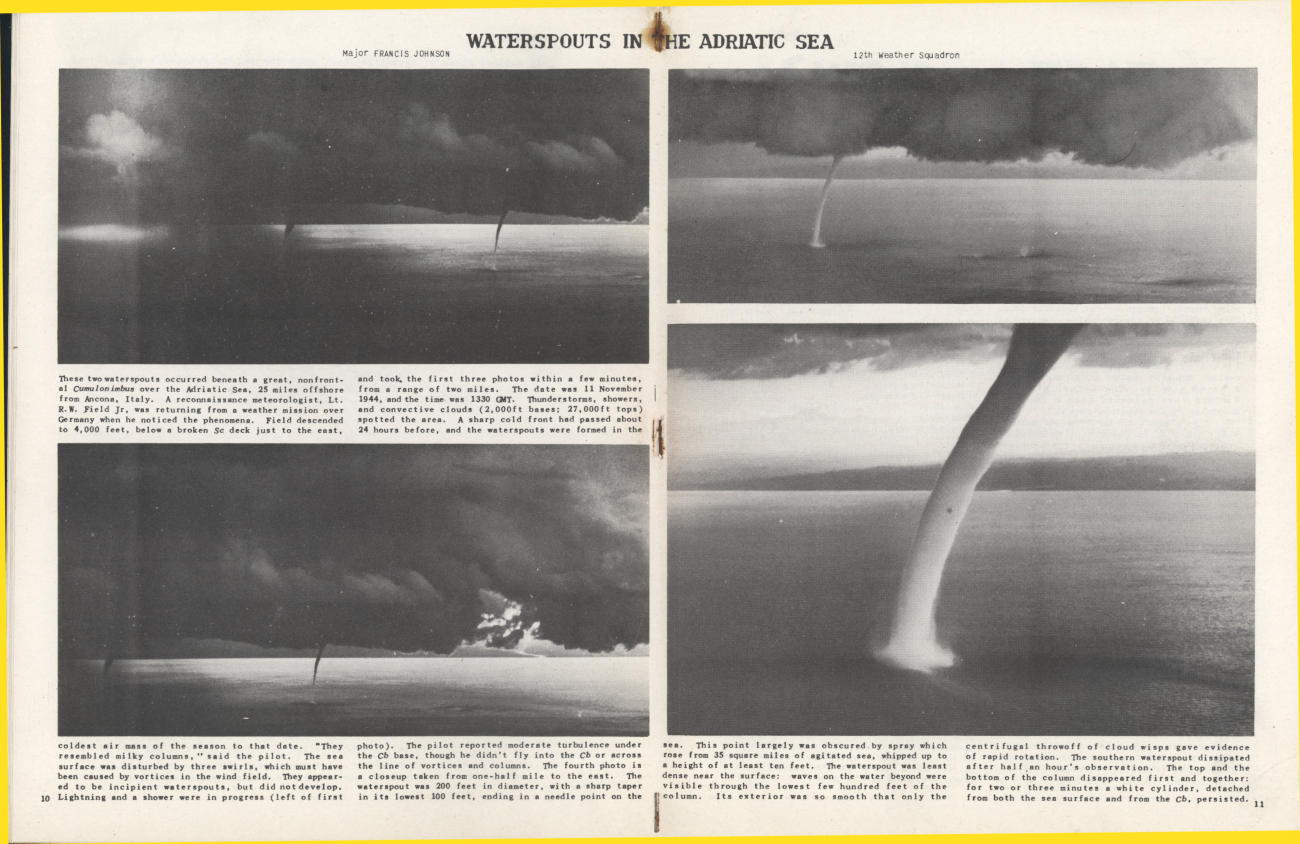This is a scan of pages 10 and 11 from a vintage book or newspaper article titled "Waterspouts in the Adriatic Sea" by Major Francis Johnson of the 125th Weather Squadron. The two-page spread features four black and white photographs with descriptions of two waterspouts. The images were captured beneath a great non-frontal cumulonimbus cloud over the Adriatic Sea, 25 miles offshore from Ancona, Italy. The photographs were taken by Lieutenant R.W. Field Jr., a reconnaissance meteorologist, who was returning from a weather mission over Germany on November 11, 1944, at 1330 GMT.

The article provides a detailed account of Field's observations. He descended to 4,000 feet below a broken stratocumulus deck just east of the phenomena and took three of the photos within a few minutes from a range of two miles. Thunderstorms, showers, and convective clouds with bases at 2,000 feet and tops at 27,000 feet dotted the area. The waterspouts, described as milky columns, formed in the coldest air mass of the season following a sharp cold front that passed 24 hours earlier. 

Field reported moderate turbulence under the cumulonimbus base, though he did not fly into it or cross the line of vortices and columns. The fourth photograph is a close-up taken from half a mile to the east, showing a waterspout that was 200 feet in diameter with a sharp taper in its lowest 100 feet, ending in a needle point on the sea. The sea surface was noticeably disturbed by three swirls likely caused by vortices in the wind field. The spray from these swirls rose from an agitated sea, where waves reached at least 10 feet high. The southern waterspout dissipated after half an hour, with the top and bottom of the column disappearing first, leaving a white cylinder briefly detached from both the sea surface and the cumulonimbus cloud.

The text is typed in a typewriter-like font, indicating its age, and the pages have a yellow and black border, further enhancing the vintage appearance.